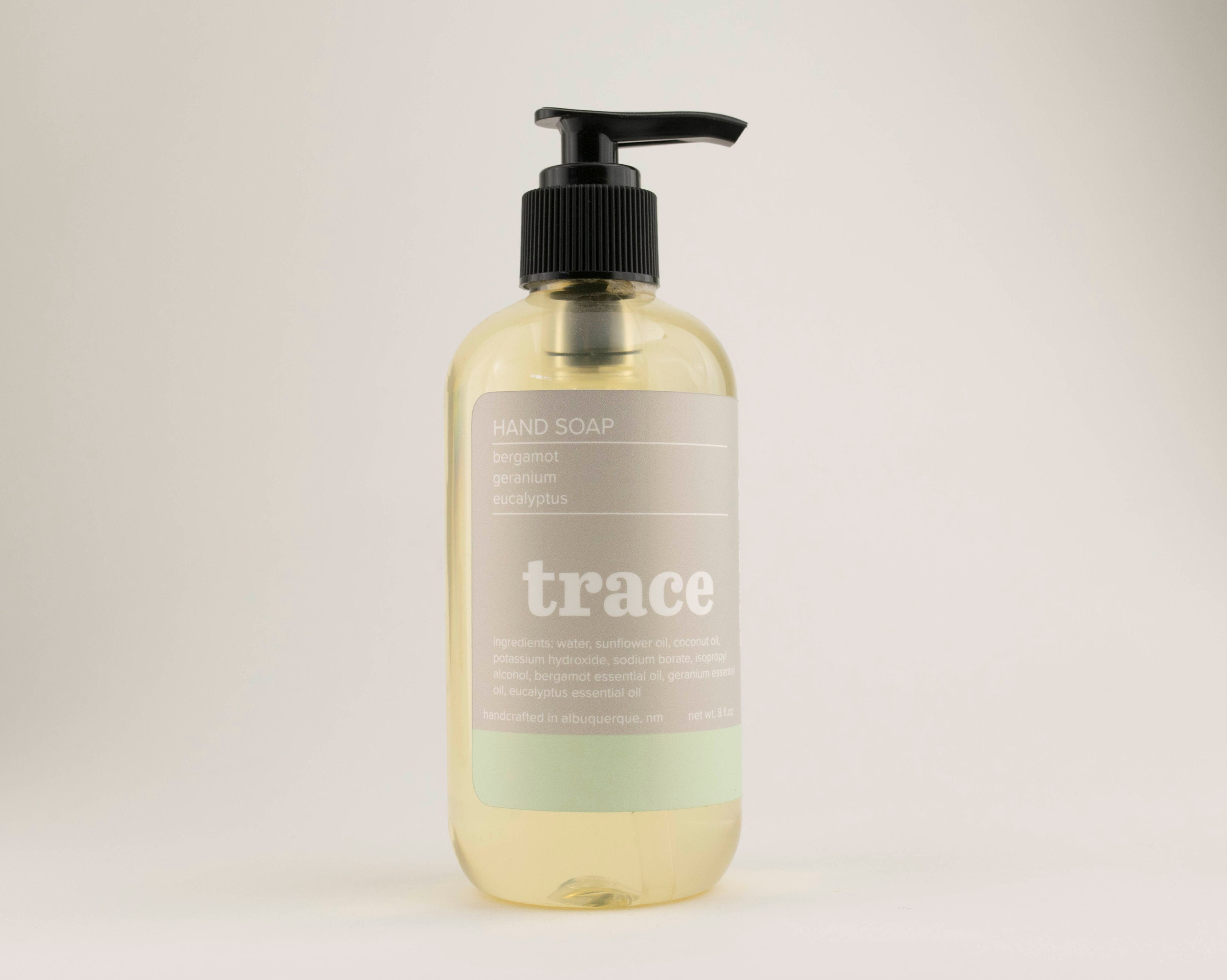This image features a modern, stylish bottle of hand soap branded "Trace." The soap is a clear, pale yellow color and comes in a round, pill-shaped bottle with a black pump handle that appears unused and is oriented to the right. The label is predominantly beige with a purplish-brown hue and a light green layer at the bottom. The text on the label is in white and details the soap's key ingredients, which include bergamot, geranium, and eucalyptus essential oils. Additional information on the label states that the soap is handcrafted in Albuquerque, New Mexico, and lists ingredients such as water, sunflower oil, coconut oil, potassium hydroxide, and sodium borate. The bottle is the sole subject of the composition, set against a plain, light purple background that suggests a photo studio setting, making it appear as though it's an advertisement for the product.